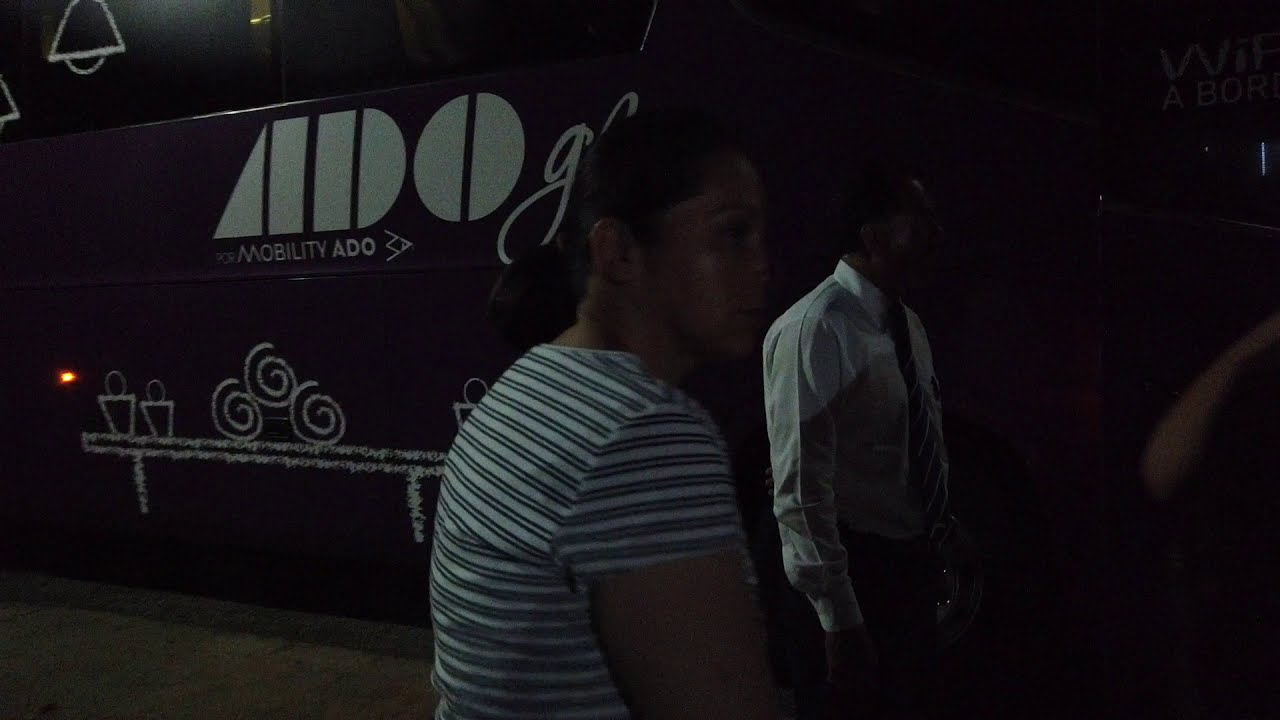This dimly lit, indoor color photograph captures a moment featuring two individuals standing side-by-side, both gazing to the right as though observing something outside the frame. At the forefront stands a woman with dark hair pulled back in a ponytail, clad in a short-sleeved, white and black striped t-shirt. Beside and slightly behind her is a man dressed in a button-up white shirt and a black and white striped tie, his face obscured by the shadows. The overall scene is shrouded in darkness, suggesting the photo might be taken at night with artificial illumination casting shadows from the upper left side of the frame. 

The pair appears to be standing in front of a large structure, possibly a bus or a wall, which features the text "ADO Mobility ADO" along with several stylized white designs that include swirls, circles, and human figures. The background has a dark purple hue, enhancing the shadowy atmosphere of the image. Glass windows are visible at the top, indicating the setting could be alongside a charter bus designed for long-distance travel. The image includes a few indistinct figures on the far right edge, further contributing to the overall scene.